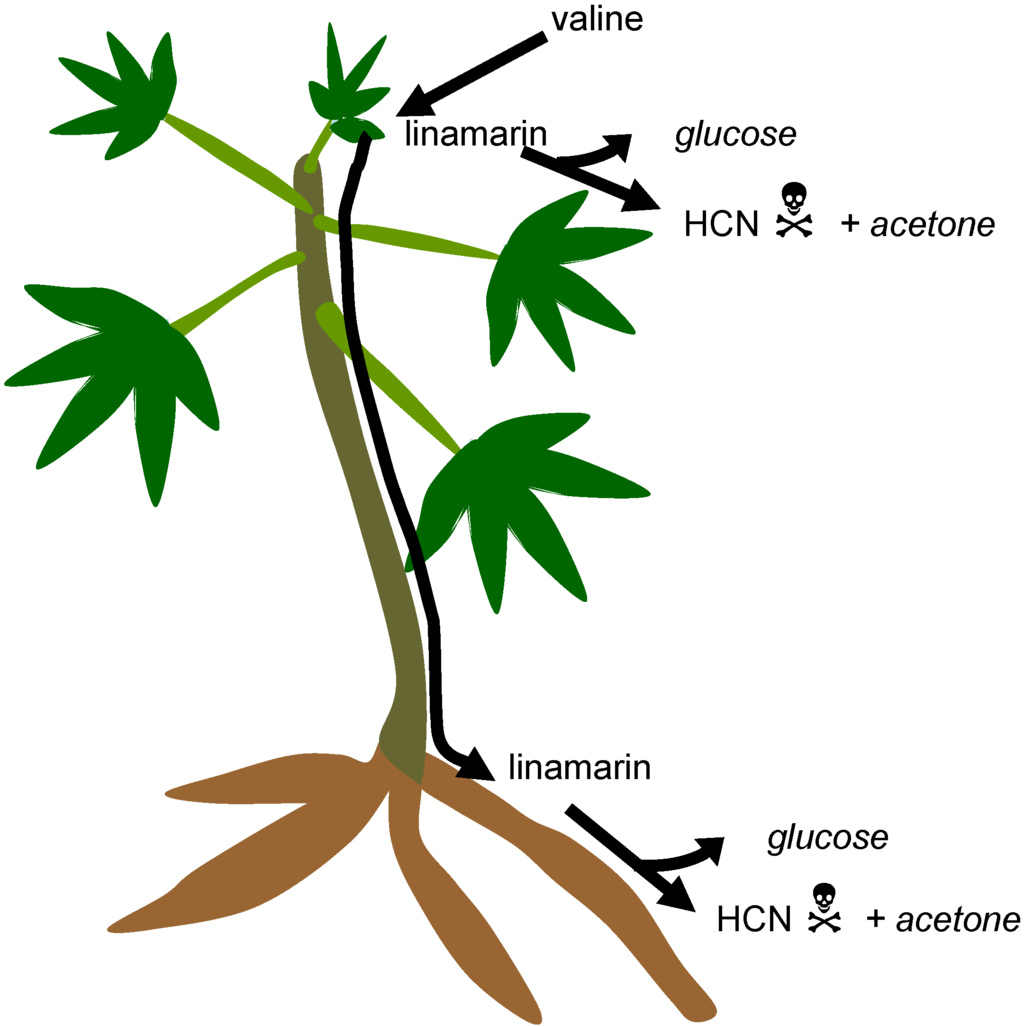The image is a detailed, hand-drawn yet computer-generated cartoon diagram of a chemical process involving a plant, presented on a white background and in portrait orientation. The plant consists of a single olive-green stalk, five light green stems, each with a medium green leaf made up of five segments, and simple brown lines indicating roots. On the right side of the plant, there is a flowchart marked entirely in black text and arrows. The flowchart starts from the word "valine" pointing to "linomerin," which then branches out with arrows leading to "glucose" and "HCN," the latter accompanied by a skull and crossbones plus the word "acetone." Additionally, "linomerin" reappears near the roots with the same branching arrows indicating "glucose" and "HCN" with the skull and crossbones plus "acetone." This setup suggests an educational visualization of the biochemical pathways involving valine, linomerin, glucose, and HCN in the plant.